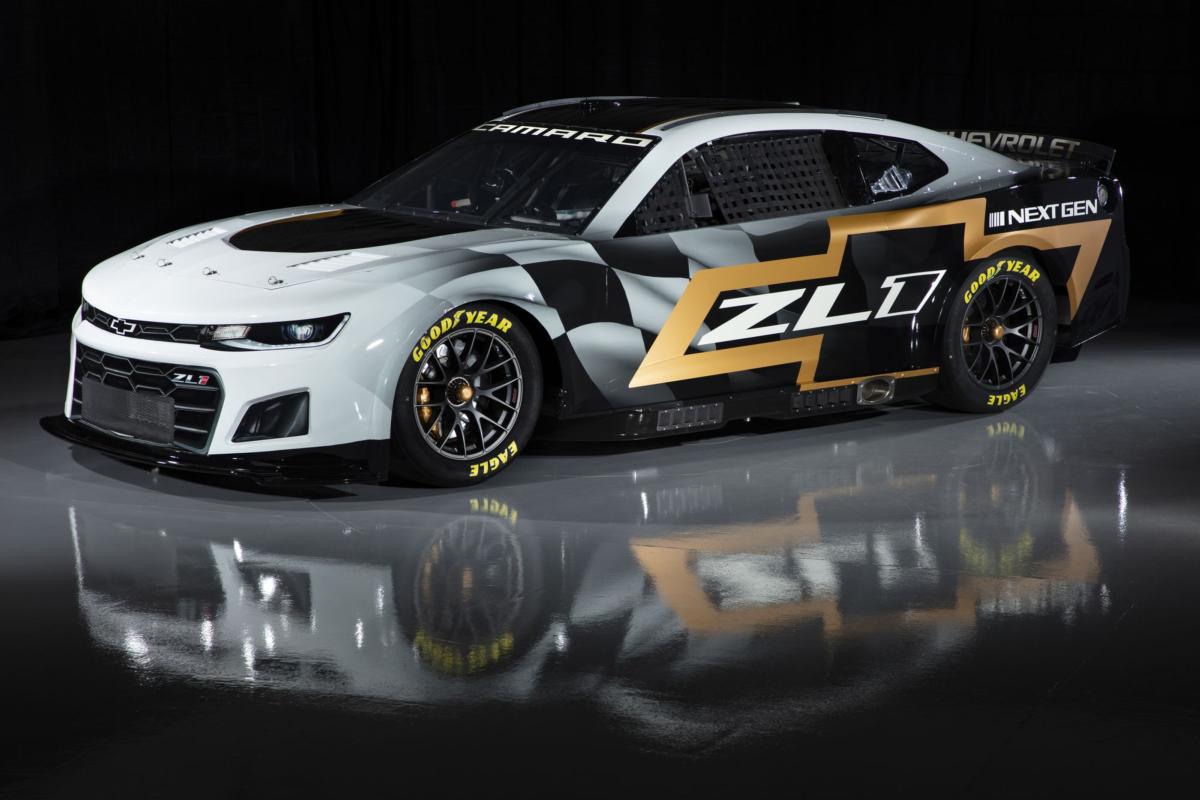This image captures a Chevrolet Camaro ZL1 NASCAR Next Gen race car, prominently displayed in a professional showroom with a reflective, mirror-like floor. The car's paint job transitions from white at the front to a combination of gray and black, accented by a bold, gold Chevrolet logo on the side. The rear of the vehicle bears the "Next Gen" designation, highlighting its modern upgrades, including wheels with a single central lug nut. The tires are branded Goodyear Eagle. The front windshield features "Camaro" prominently, reinforcing the model, while the side showcases "ZL1" in white letters. The background is completely black, enhancing the focus on the car and its detailed reflection on the shiny floor. The sleek design, professional setting, and visible decals underscore its status as a cutting-edge race car built for NASCAR's Next Gen series.